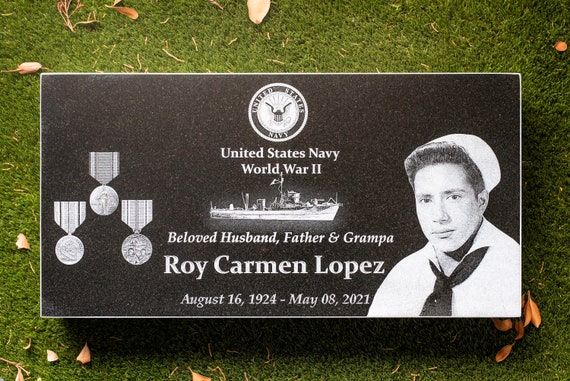This aerial photograph captures the gravestone of Roy Carmen Lopez, a World War II United States Navy veteran. The gravestone, crafted from textured granite, is intricately designed and set against a background of green grass with some dried leaves scattered around. The top portion of the rectangular headstone prominently features the United States Navy emblem, a detailed white bird within a black-bordered circle. Below this emblem, the inscription "United States Navy, World War II" is clearly visible in white text on a dark gray background.

Central to the gravestone's design is an engraved image of a Navy ship, symbolizing Lopez's service. Beneath the ship, the heartfelt tribute reads, "Beloved Husband, Father and Grandpa, Roy Carmen Lopez," followed by the dates of his birth and death, "August 16, 1924, to May 8, 2021." To the left of this text, three engraved medals are displayed, likely representing the honors Lopez earned during his naval service. On the right side, a photograph of Lopez in his Navy uniform has been etched into the stone, depicting him in a white sailor uniform with a black necktie and a white hat, clearly showing his white skin and dark hair. The entire composition reflects a fitting memorial to a respected and loved veteran.